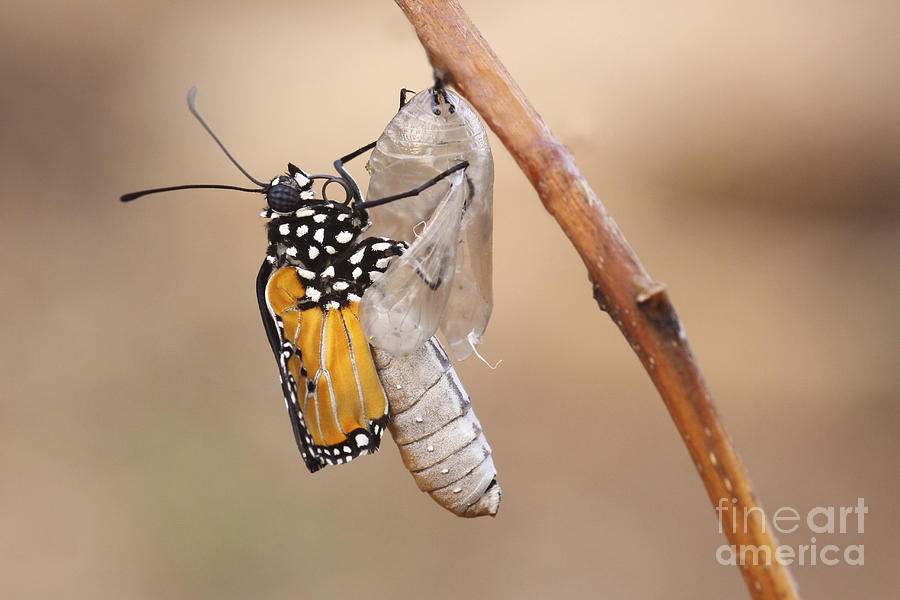The photograph captures an intricate close-up of a butterfly emerging from its cocoon, attached to a light orangey-brown twig that extends from the lower right corner to the middle top. The background is a beautifully blurred blend of tan and faint green hues, adding depth without distracting from the main subject. The butterfly, resembling a monarch with its striking yellow wings accented by black borders and white spots, is almost fully emerged, showcasing its delicate but detailed antlers and vibrant body. The cocoon, adorned with black lines, contrasts sharply against the muted backdrop, further emphasizing the transformation taking place. In the lower right corner, the text "Fine Art America" appears in clear white font, subtly branding the fine art photograph.